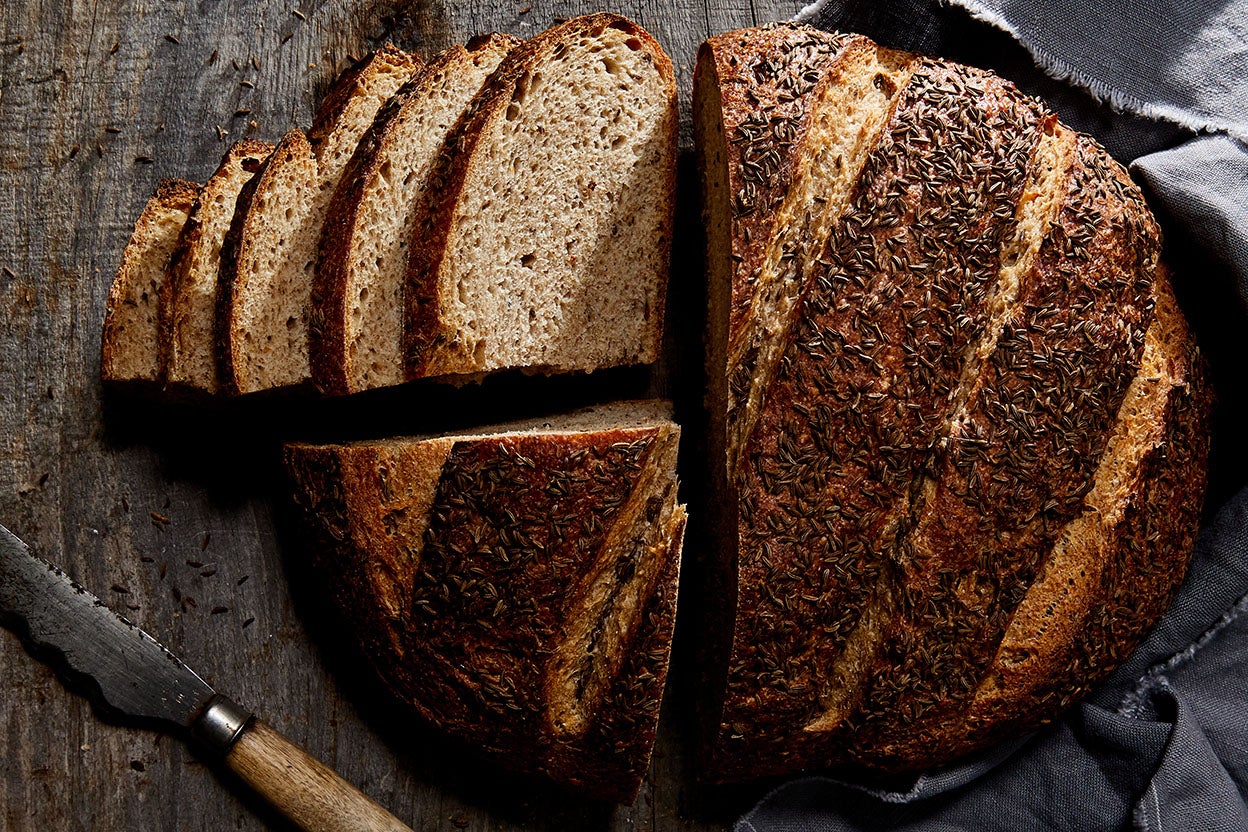This professionally-taken, color photograph features a fresh-baked loaf of bread in landscape orientation. The bread, which has a circular dome-like, oblong elliptical shape, rests on a rustic wooden table. Its crust is dark brown with diagonal slash marks of lighter brown, imparting a detailed, grainy texture. The left portion of the bread has been intricately cut: it is sliced in half, with one of those halves further divided. The top left quarter has been sliced into multiple light beige slices, while the bottom left quarter remains intact. Below, to the left of the loaf, a knife with a light wood handle and a stainless blade is positioned, partially cropped from view. The composition exudes a photographic realism style, showcasing food photography at its finest.